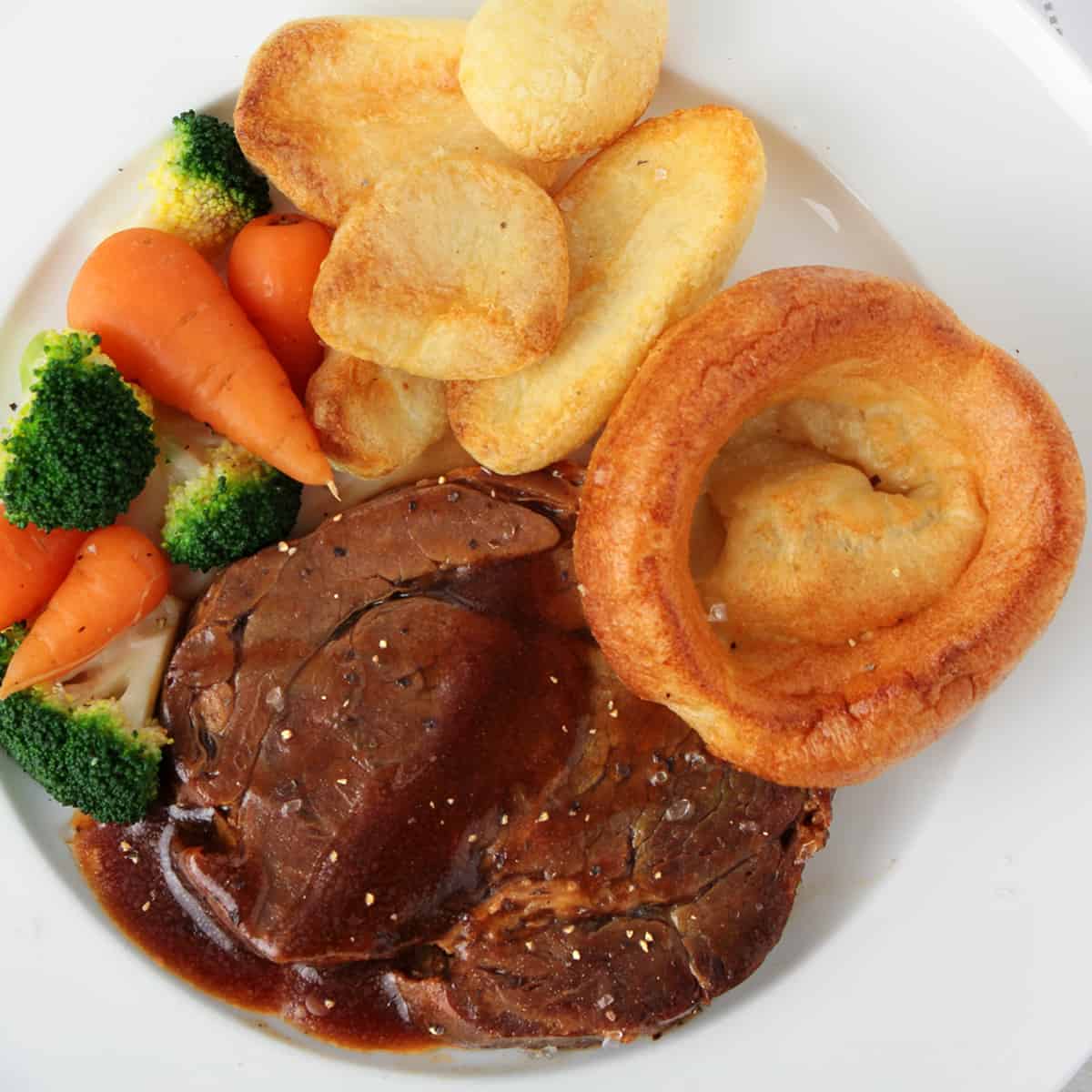On a small, spiral white plate, there is a meticulously arranged variety of foods. At the bottom center, a generous piece of prime rib is adorned with a creamy gravy, sprinkled with parsley, salt, and pepper granules. To its left, at the 9 o'clock position, lie several baby carrots and broccoli florets, vividly colored and neatly presented. To the right of the steak is a round, soft-centered item with a darker edge, potentially a bread pudding. Additionally, there are small bread bites on the opposite end of the plate. A slight spill of gravy extends from the steak towards the plate's edge, and the plate's intricate shadow reveals its indented center, although the direction of the light source is indiscernible from the image.